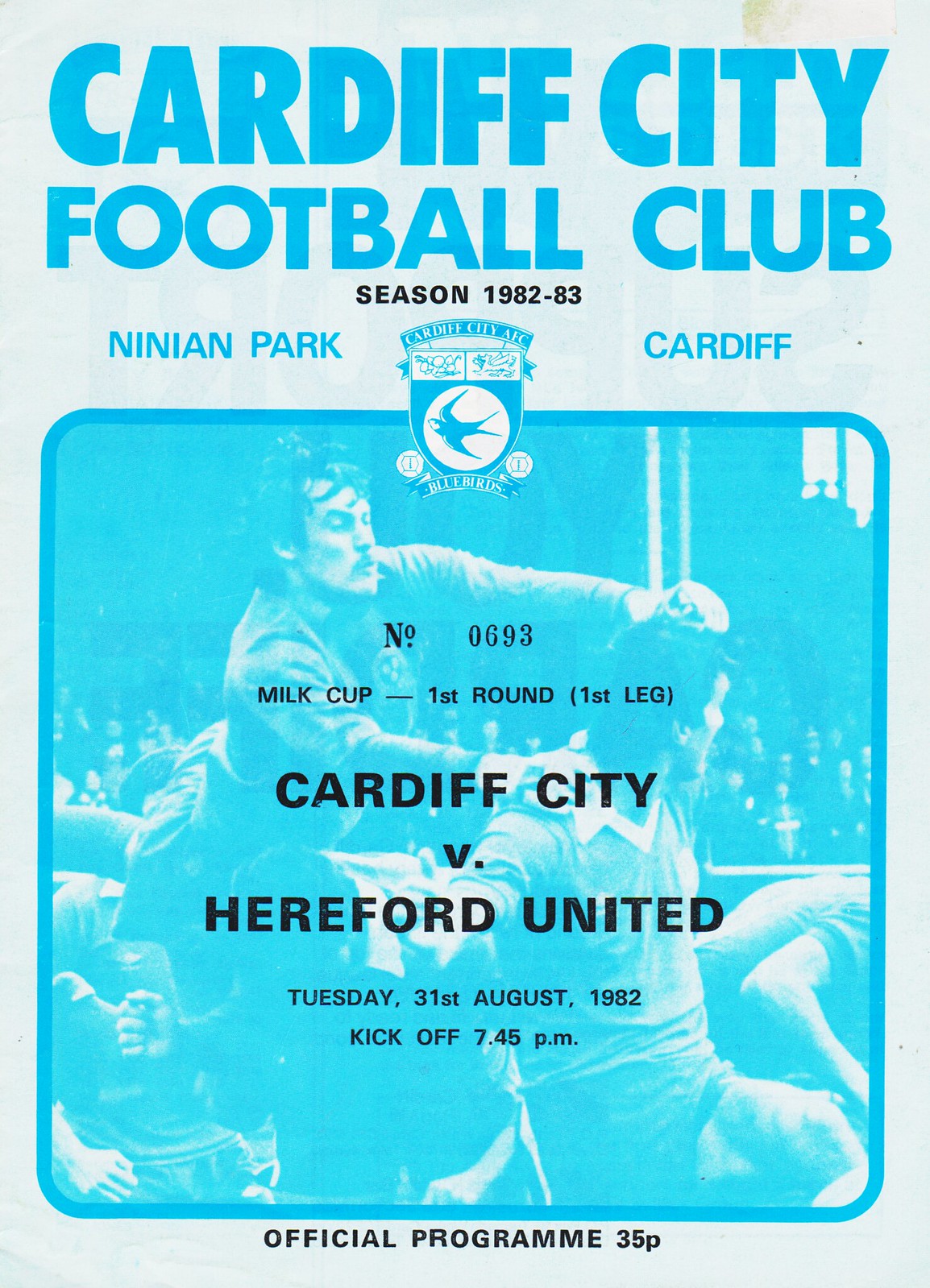This detailed image description combines elements from both voice descriptions, highlighting shared and repeated details. 

---

The image is a cover of what appears to be an official matchday program from 1982. The background of the rectangular poster is primarily a light green color. Dominating the lower section of the cover is a tinted blue photograph depicting a dynamic action scene where one soccer player seems to be diving into another, with several people visible sitting in the background. Overlaid on this photograph, in black text, is the inscription: "No. 0693 Milk Cup - First Round (First Leg) - Cardiff City vs. Hereford United - Tuesday, 31st August 1982, Kick-off 7:45 PM."

At the top of the image, text in blue reads: "Cardiff City Football Club Season 1982-83, Ninian Park, Cardiff." Positioned between these blue letters is the club’s crest, featuring a shield with a bird and the words "Cardiff City AFC - Bluebirds." At the very bottom of the cover, the text "Official Program 35p" appears, solidifying its authenticity. The cohesive use of blue and green hues, along with the well-distributed text and imagery, presents a visually appealing and informative cover for the historical event.